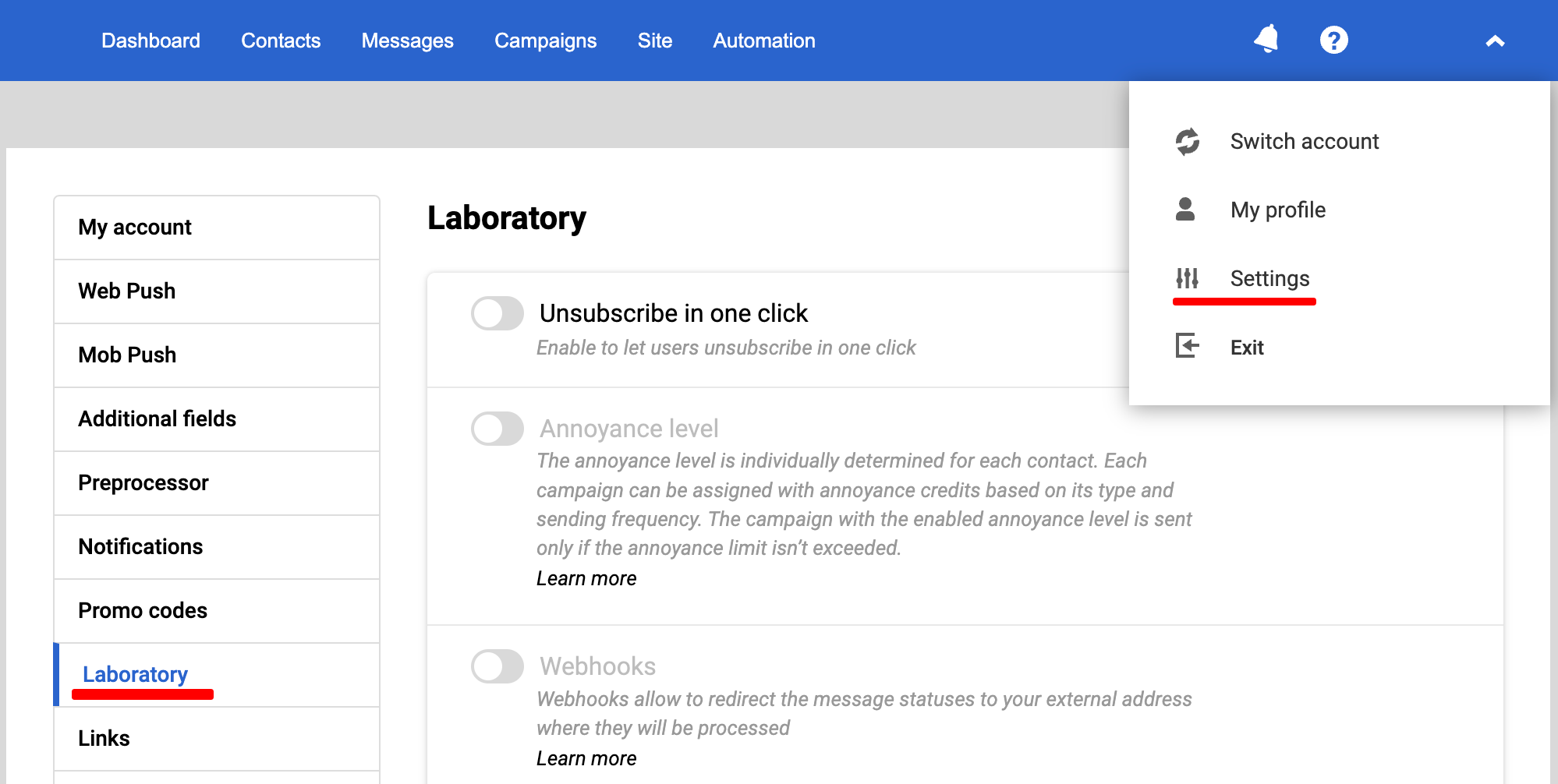This image shows a computer screen with a user interface primarily dominated by a royal blue toolbar at the top. The toolbar spans the width of the screen and features several sections labeled in white text: "Dashboard," "Contacts," "Messages," "Campaigns," "Site," and centrally located "Automation." To the right of these sections, there's a white notification bell icon, a white circle containing a blue question mark, and an upward-pointing arrowhead.

Beneath this blue toolbar, a grayscale bar of equal width stretches across the screen. Below this bar, the main content area is presented on a white background. At the top of this section, the word "Laboratory" is prominently displayed in black letters. Below "Laboratory," three distinct sections each featuring a toggle switch are organized vertically.

1. The first section, labeled "Unsubscribe in one click," includes a toggle switch (ellipse with a white circle and a gray semicircle to the right) and a line of smaller text below that reads, "Enable to let users unsubscribe in one click."
2. The second section, labeled "Annoyance level," also features a toggle switch and a paragraph of text approximately five to six lines long, ending with a bolded "Learn more."
3. The third section, titled "Webhooks," includes a similar toggle switch with two lines of descriptive text stating, "Webhooks allow to redirect the message statuses to your external address, where they will be processed." Like the second section, it finishes with a bolded "Learn more."

To the left of the main content area, there is a sidebar menu with nine rows of items separated by faint gray lines. Each item is titled in black text, except for "Laboratory," which is highlighted in blue and underlined with a thick red line. There’s also a blue vertical line to the left of "Laboratory." The sidebar menu items are listed as follows: "My Account," "Web Push," "Mob Push," "Additional Fields," "Preprocessor," "Notifications," "Promo Codes," "Laboratory," and finally "Links."

An open dropdown menu under the notification area on the right side includes four rows, each with an icon and text:
1. A circular arrow icon alongside "Switch account" in gray text.
2. An icon of a person next to "My profile."
3. An unidentified icon resembling three vertical lines, adjacent to "Settings," which is underlined with a red bar.
4. A gray square missing the right-hand side, with an inward-pointing arrow, next to "Exit."

The detailed layout presents a comprehensive snapshot of the user interface, covering multiple functionalities and options available within the application.